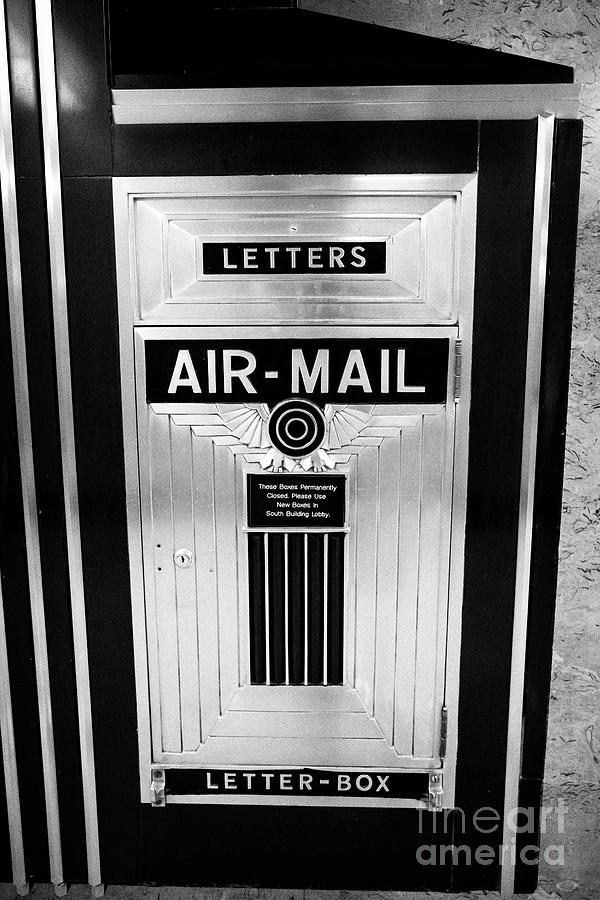This black-and-white photograph captures a vintage mailbox, likely from the 1920s to 1960s, embedded in what appears to be a marble or granite wall. The mailbox, designed in an art deco style, features a black lacquered or dark metal front with silver accents and trim. At the top of the box, there is a slot labeled "LETTERS" in bold, white, capitalized letters on a black background. Below this slot is a door with a lock, which the postman would use to retrieve the mail. The door displays the words "AIR MAIL," also in white letters on a black background, beneath which is a circular emblem resembling pilot's wings. Additional unreadable text follows, and at the very bottom of the door, the word "LETTERBOX" is inscribed in a black banner. The entire mailbox has vertical stainless steel-like designs. In the bottom right corner of the image, there is a watermark that reads "Fine Art America."